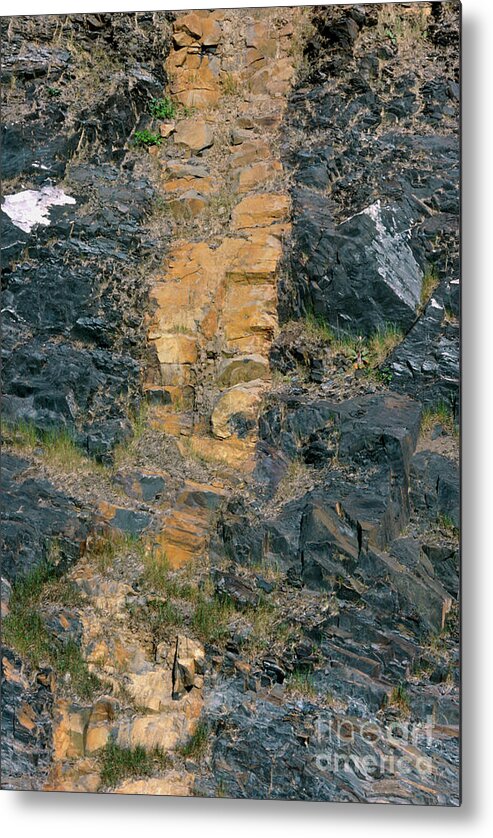The image is a close-up, highly detailed view of a rocky landscape, possibly a painting or a photograph, displayed as framed art that you might hang in a home or office. The focal point of the image is a rugged, rocky surface with a distinct vertical streak of brown, orange, or clay-colored material running through the middle, which narrows toward the top. This central stripe slightly veers to the left and is interspersed with small patches of greenery—grasses, moss, or weeds—throughout. Black rocks flank both sides of this central strip, showing variation in texture from jagged to smooth edges. In the upper left corner, a white patch, possibly snow or a different type of rock, adds contrast to the predominantly earthy tones. The bottom right contains some hard-to-read text that appears to reference art and America, potentially reading "ripe art America." The image's scale and perspective are ambiguous due to the zoomed-in view, making it challenging to discern whether it depicts a real landscape or an artistic rendition.